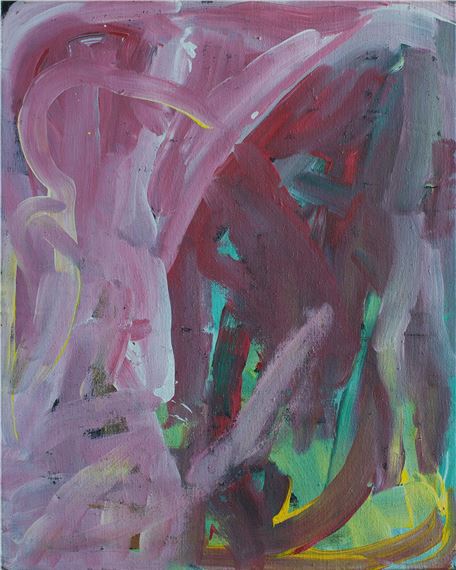This is an abstract painting featuring broad, dynamic brush strokes primarily moving up and down with some diagonal and swirling patterns. The left half of the canvas is dominated by varying shades of purple, from light to dark, interspersed with grays. The right side transitions into deeper hues, including rich reds, while incorporating teal, yellow, and hints of blue. The lower right corner introduces a few brown swirls highlighted in golden yellow, suggesting a concentrated source of light. The central area showcases saturated pinky-gray tones, contributing to the painting's overall texture and depth. Some elements evoke a watery, coral-like scene, with intertwining tube-like forms reminiscent of oceanic coral structures, adding a sense of underwater serenity. The entire composition is saturated and dense, with a watercolor effect despite being rendered in oils or acrylics.